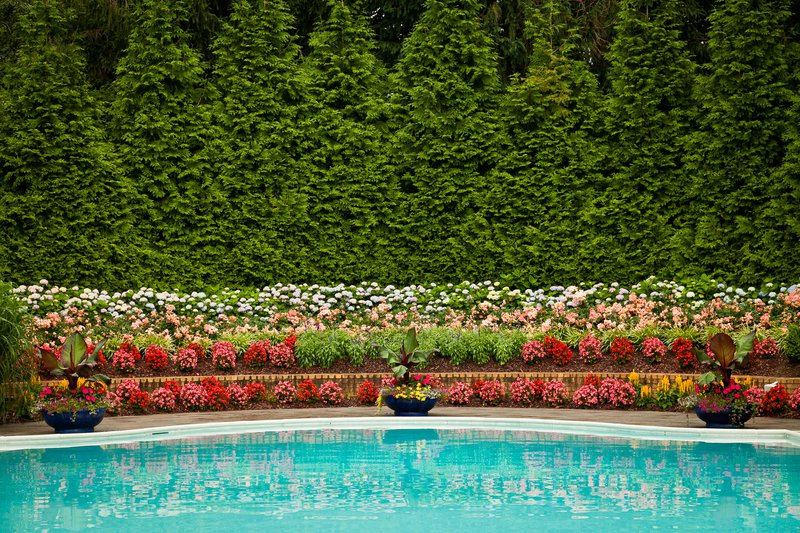This realistic photograph, horizontally oriented and text-free, captures an outdoor daytime scene dominated by lush greenery and vibrant flora. In the foreground, a pristine pool with crystal clear, bright blue water is framed by a white-edged border and a gray cement pool deck. Three black potted plants with vivid blooms—red flowers on the left, yellow in the center, and red again on the right—add a touch of elegance to the poolside.

Moving back from the pool deck, the garden is tiered, creating a visually appealing formal arrangement. The lower tier features a row of vibrant red and pink small flowers, while the middle tier showcases a mix of pink and red circular rose bushes. The upper tier is adorned with a row of light pink roses, followed by a tier of white roses at the highest level. Each tiered floral arrangement adds depth and color to the scene.

Dominating the entire upper half of the image are tall, lush evergreen trees that form a dense, hedge-like backdrop, effectively blocking any view of the sky and enhancing the garden's serene, secluded ambiance. This harmonious blend of water, flora, and greenery creates a tranquil, picturesque setting.